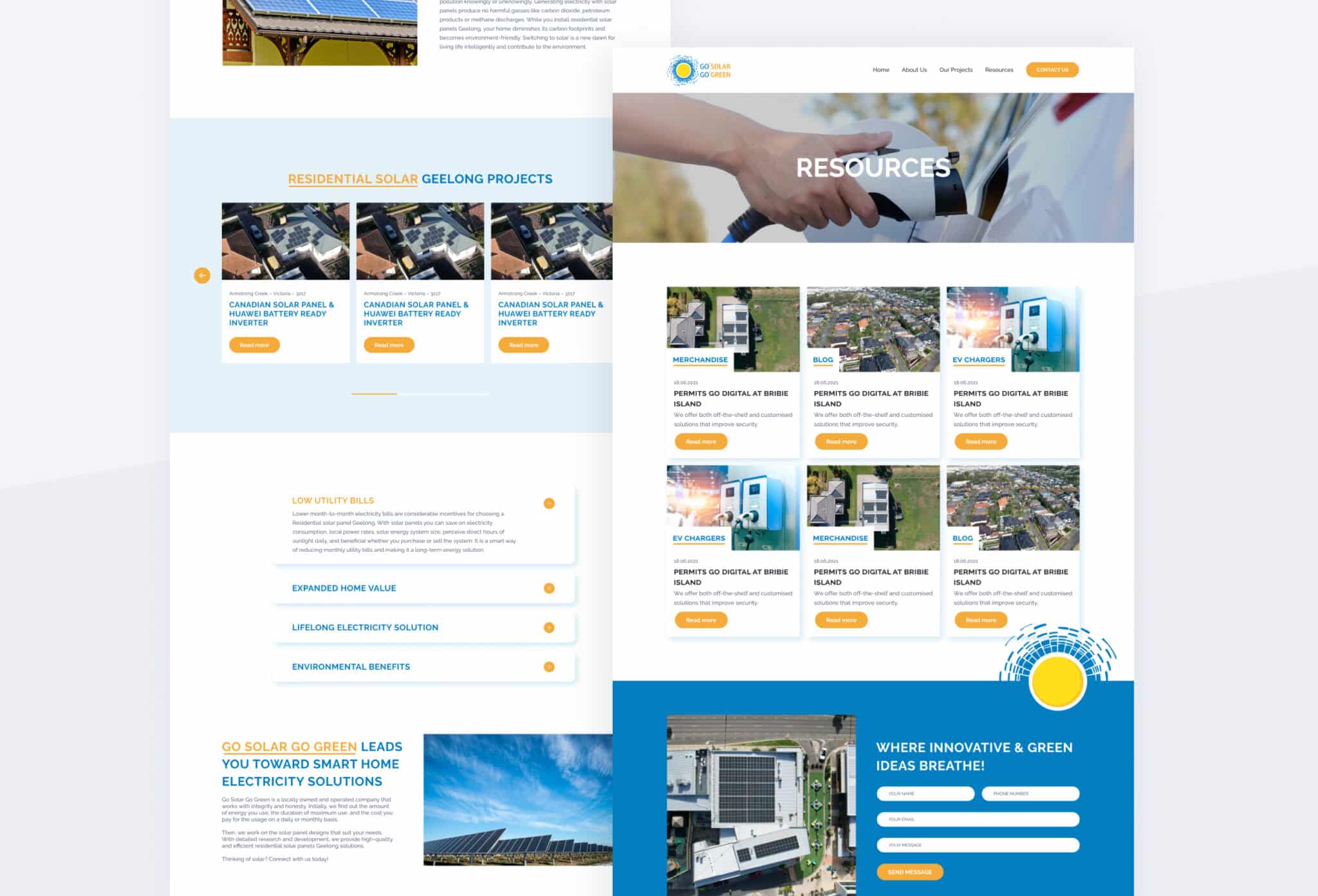A detailed screenshot of a promotional website advocating for solar energy usage. At the top left corner, the phrase "Residential Solar" is prominently displayed in underlined orange text, followed by "Geelong Projects" in blue text. Below this header, there are various articles listed, including titles like "Canadian Solar Panel" and "Huawei Battery Ready Inverter." Interestingly, the content of these two articles appears to be identical and somewhat redundant. Beneath these listings, there are several tabs highlighting the benefits of solar energy, labeled "Low Utility Bills," "Expanded Home Value," "Lifelong Electricity Solution," and "Environmental Benefits." To the right side of the page, a section titled "Resources" is visible, featuring multiple articles with titles such as "Permanent Scope Digital at Bird Bridge Island," each accompanied by different images but sharing the same content. The entire layout emphasizes the advantages and positive impact of adopting solar energy over traditional energy sources.